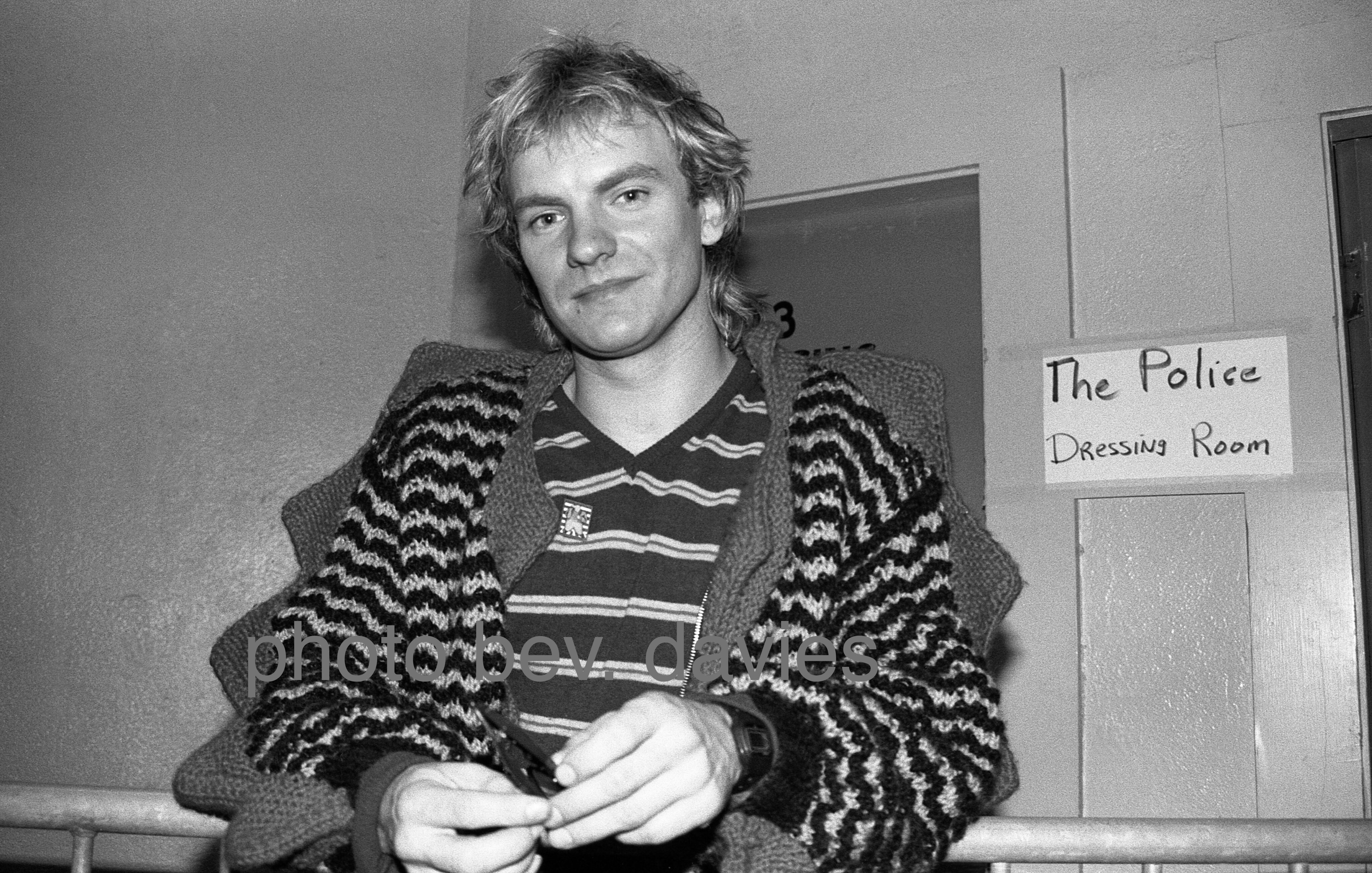This is a black and white photograph featuring Gordon Sumner, famously known as Sting, during his tenure with the band The Police. Sting, a Caucasian male with slightly messy, short-to-medium length blonde hair, is captured wearing a distinctive outfit consisting of a fuzzy, black and white striped knitted sweater with spiky textures and a striped v-neck t-shirt underneath. He is slightly smirking at the camera with his hands gently touching each other. In the backdrop, a handwritten sign on a concrete wall reads "The Police Dressing Room," indicating a likely backstage setting. The image, marked with a Photo Bev Davies watermark in sans-serif font, portrays a candid moment before a performance, depicting Sting's relaxed demeanor. The room also features a railing he is leaning on and two doors, adding to the backstage ambiance.